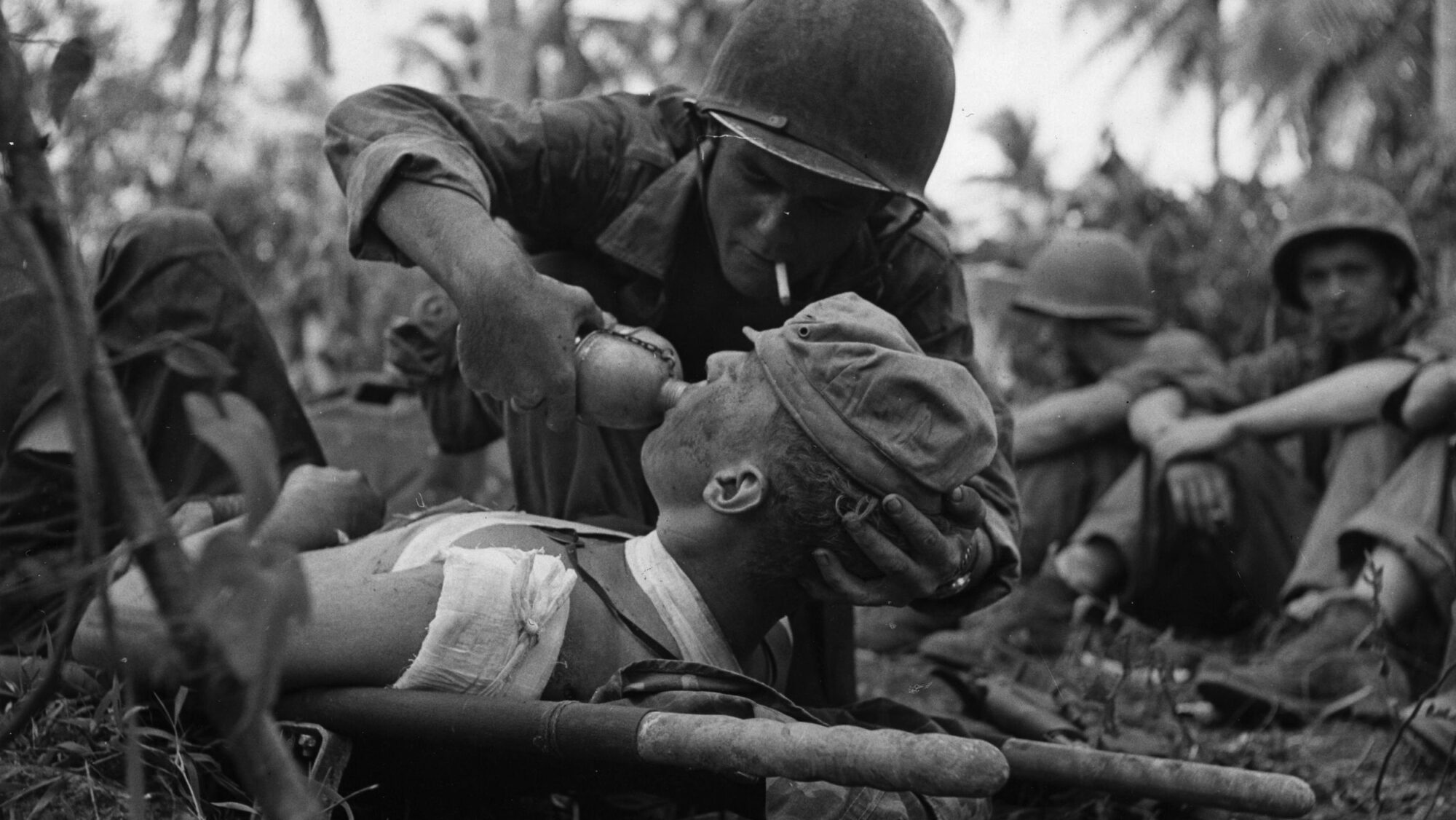In this black and white wartime photograph, likely from the Vietnam War given its jungle setting, several soldiers in combat fatigues and helmets occupy a clearing surrounded by trees and vegetation under a bright sky. At the center of the image, a soldier, with a cigarette in his mouth and wearing a helmet, crouches over an injured comrade who lies on a stretcher. The injured man, distinguishable by his cap and white undershirt, has a bandaged shoulder in a sling and dirt on his face. With one hand, the helmeted soldier steadies the injured man's head, while with the other, he pours water from a metal canteen into his mouth. To the right side of the image, three more soldiers are visible, seated on the ground with knees up and arms resting on them, their gazes directed toward the central figures. This poignant scene, capturing a moment of care amidst the chaos, evokes the harsh realities of war.